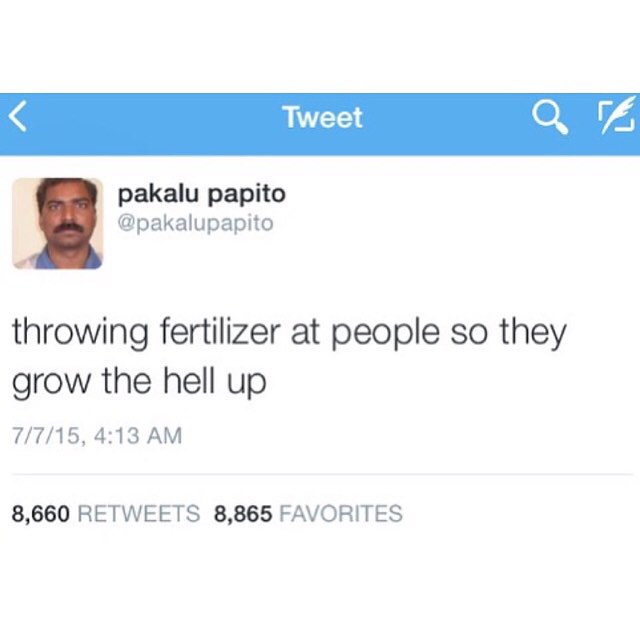The image is a detailed screenshot of a tweet from the popular Twitter account Pakalu Papito. At the top, the classic Twitter blue bar is visible, featuring menu options like 'Tweet,' 'Back,' and a search icon. Below this banner, the tweet displays a self-portrait of a Mexican man named Pakalu Papito, who has short brown hair and a mustache, and is dressed in a white shirt with a blue collar. His tweet humorously states, "Throwing fertilizer at people so they grow the hell up." This post was made on July 7, 2015, at 4:13 AM. It garnered significant engagement, with 8,660 retweets and 8,865 favorites.